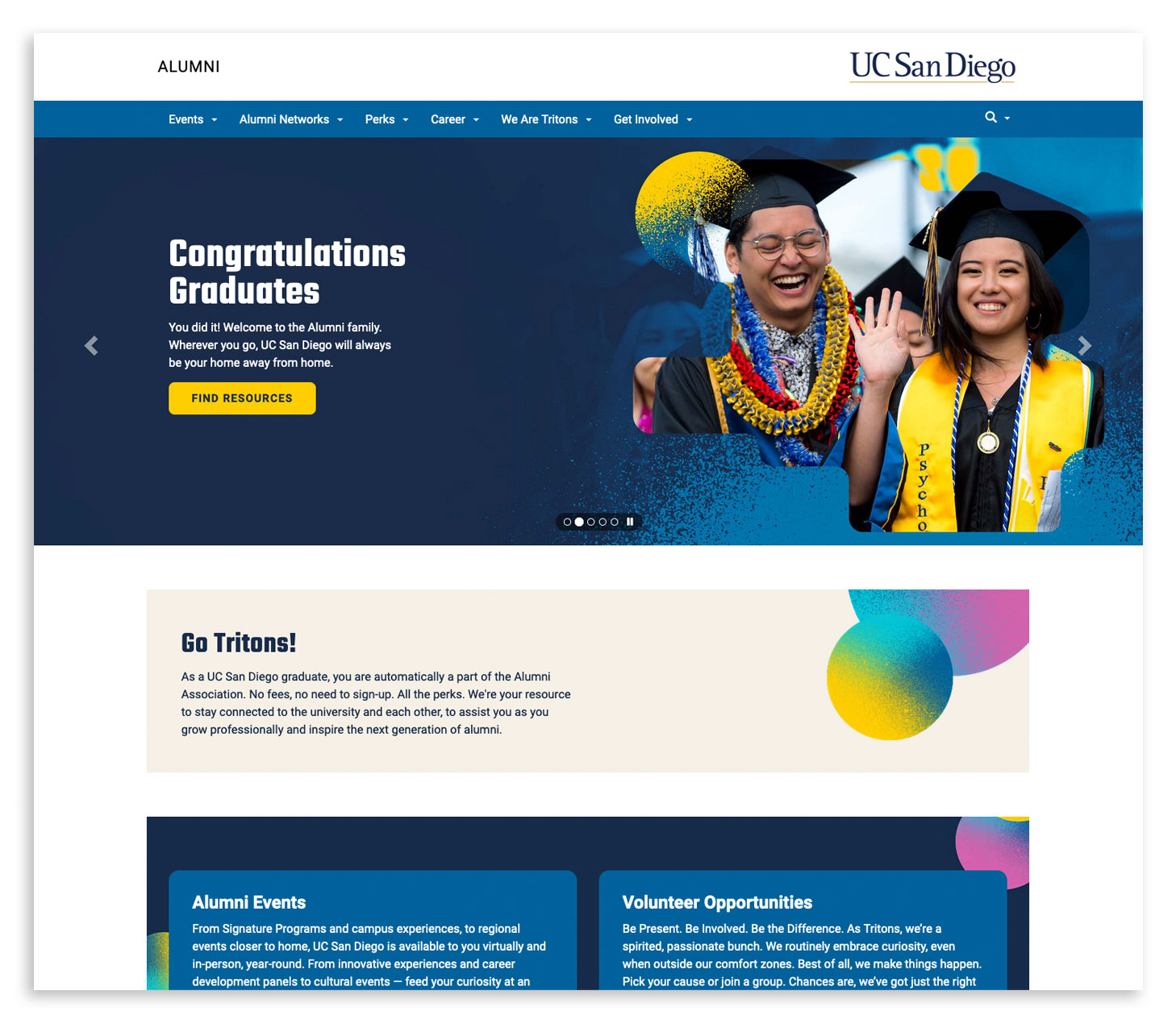The image depicts a section of a web page featuring a celebratory theme for graduates. At the top, there is a clean white banner. On the far left, in small black capital letters, is the word "ALUMNI." Towards the right side of the banner, the text "UC San Diego" appears in a dark blue font, with "S" and "D" capitalized and underlined. Below this, a search bar is visible.

Directly under the white banner, a thin light blue bar spans the width of the page. It contains several clickable dropdown menus labeled: "Events," "Alumni Networks," "Perks," "Career," "We Are Tritons," and "Get Involved." 

Beneath the light blue bar, bold white text on the left reads, "Congratulations Graduates!" followed by "You did it, welcome to the alumni family. Wherever you go, UC San Diego will always be your home away from home." Adjacent to this congratulatory message is a prominent gold button with the text "Find Resources" in blue, indicating further information can be accessed by clicking on it.

To the right of this text block, there is an image of a joyous graduating duo: a man and a woman dressed in their academic regalia. The woman has her hand raised in a celebratory gesture, while the man appears thrilled and content. They embody the excitement and relief of graduation.

Below this main section, there are navigational arrows on the left and right sides, allowing users to scroll through additional content. Underneath these components, phrases like "Go Tritons," "Alumni Events," and "Volunteer Opportunities" are displayed, highlighting further engagement opportunities for alumni.